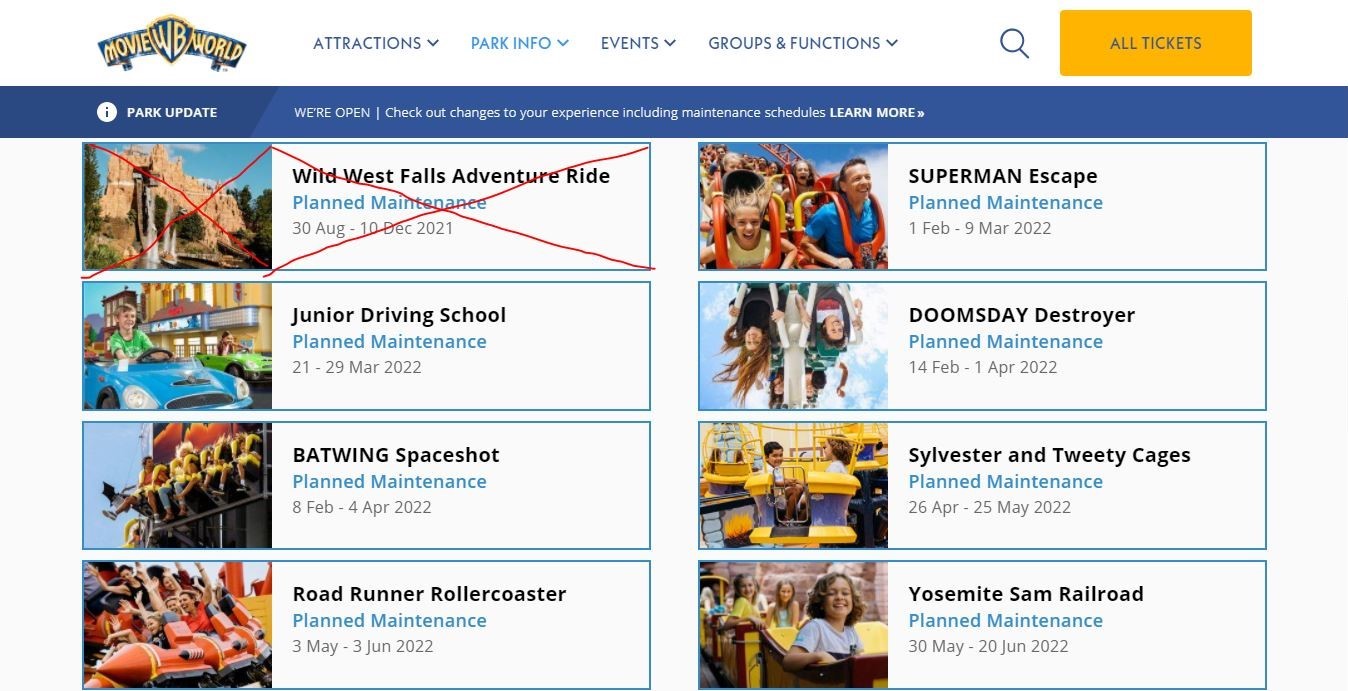This screenshot captures the retro aesthetic of the Warner Brothers' MovieWorld website, likely from the early 2000s. Dominating the top left corner is the iconic MovieWorld logo, accompanied by the timeless Warner Bros. shield logo. To the right, there are four drop-down menus labeled "Attractions," "Park Info," "Events," and "Groups and Functions," each featuring a downward arrow indicating more options. Next to these menus, a sleek search bar and magnifying glass icon are positioned, along with a prominent gold rectangular button labeled "All Tickets."

Beneath this navigational bar is a headline reading "Park Update." The update informs visitors that the park is open and encourages them to check out changes to their experience, including maintenance schedules, with a prompt to "Learn More." 

Further down, the page showcases a collection of rides with small accompanying images. These rides include the "Wild Wild West Falls Adventure Ride," "Superman Escape," "Doomsday Destroyer," "Junior Driving School," "Batwing Space Shot," "Sylvester and Tweety Cages," "Roadrunner Roller Coaster," and the "Yosemite Sam Railroad." Each ride is depicted with a thumbnail image, enhancing the viewer's anticipation and excitement.